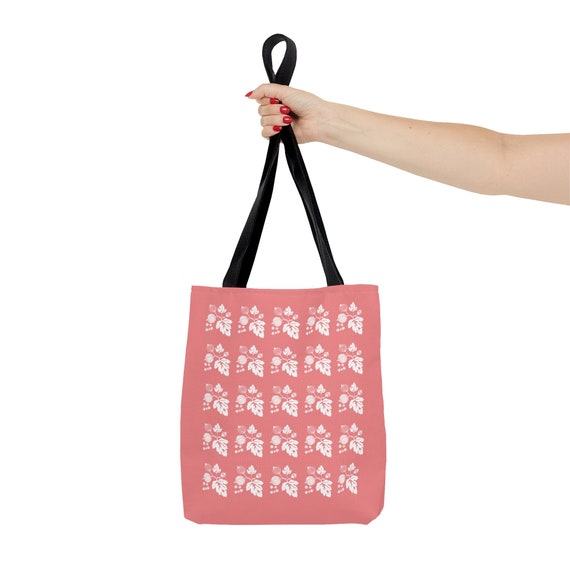In this color photograph, set against a solid white background, a woman's arm extends from the upper right, reaching out straight and ending just above the elbow. Her fingernails are painted in bright red polish, adding a splash of vibrant color to the image. She clutches a large pink tote bag by its black, material-like straps, which are crossed. The tote, reminiscent of a canvas material, showcases a meticulously arranged pattern of white floral designs. These flowers, each accompanied by a leaf, are aligned in perfect rows of five, creating a total of 25 uniform floral arrangements that appear computer-generated in their precision. The focus on the arm and tote bag highlights the detailed craftsmanship and distinct features of both elements in the photograph.